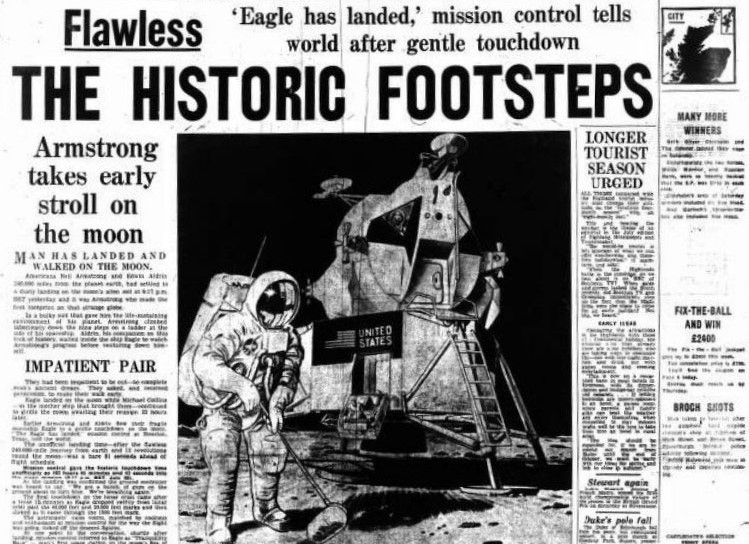The newspaper clipping in the image is a black-and-white article primarily focused on the historic Apollo 11 moon landing. At the top left, the headline reads "Eagle has landed, Mission Control tells world after gentle touchdown," followed by "Historic Footsteps." The centerpiece is a detailed drawing of an astronaut, likely Neil Armstrong, dressed in a white spacesuit standing in front of a lunar lander, with the black background of space and the grayish-white surface of the moon. Text alongside the image highlights "Armstrong takes early stroll on the moon" and "Man has landed and walked on the moon." Below, large bold letters say "Impatient Pair." Adjacent to this article, the headline "Longer Tourist Season Urged" is visible, along with other minor snippets of articles about lottery winners and city news, indicating a multifaceted newspaper layout despite the central focus on the momentous moon landing event.